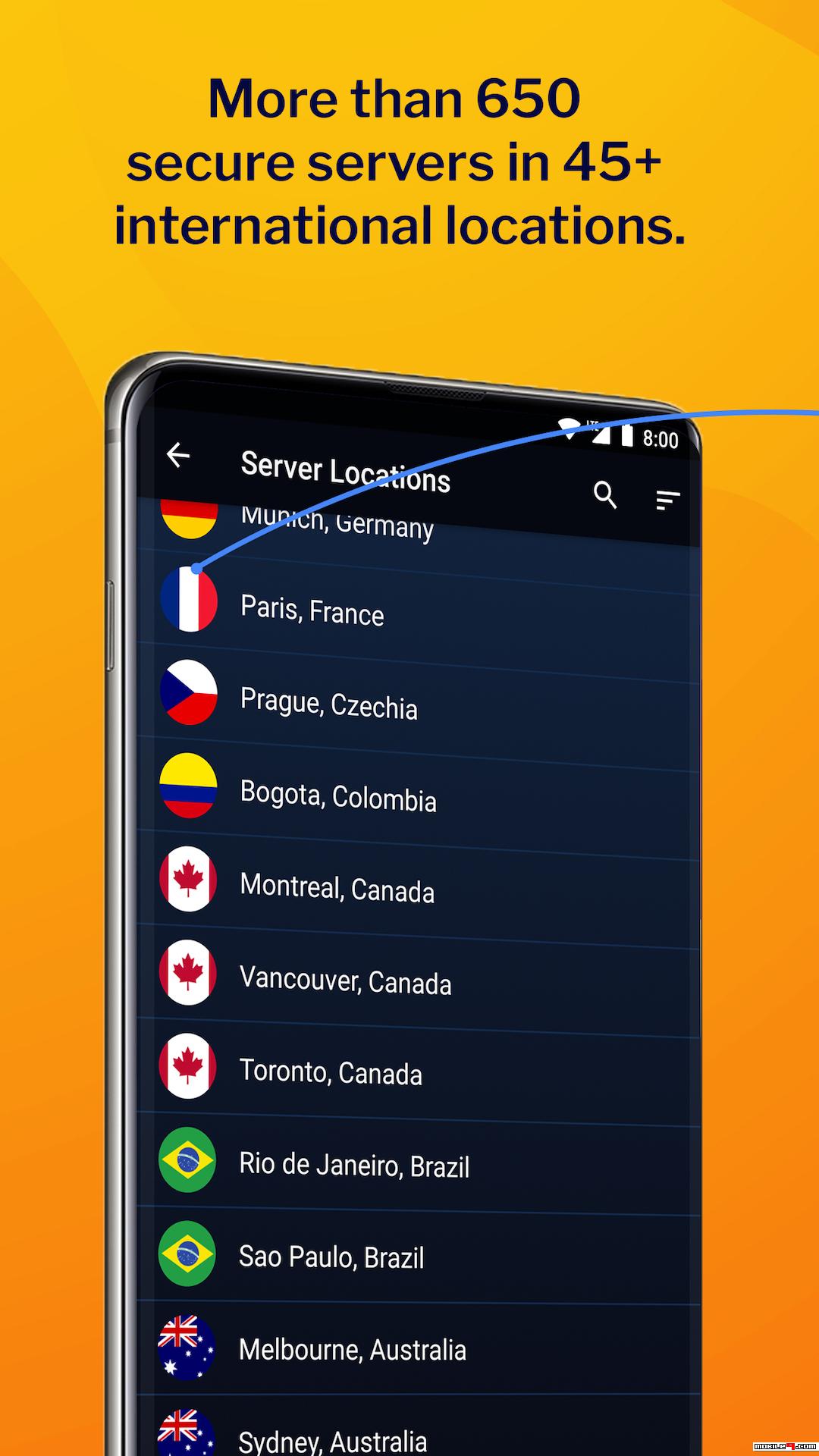The image depicts a digital advertisement with an orange background featuring two shades of orange - a lighter and a darker one. Prominently displayed in black text is the information: "More than 650 secure servers in 45+ international locations." Central to the image is a slightly angled smartphone showing various connection indicators: "APM" with full battery, full cell service, LTE, and full wireless connection. Emanating from the phone is a blue line that intersects with a circle displaying the French flag, giving an impression of connectivity extending beyond the screen.

Below the phone graphic, there's a black navigation bar featuring a back button, a text field labeled "Server Locations," a magnifying glass search icon, and a three-bar menu icon. Listed underneath this bar are server location options alongside their respective country flags: Munich, Germany; Paris, France; Prague, Czechia; Bogota, Colombia; Montreal, Canada; Vancouver, Canada; Toronto, Canada; Rio de Janeiro, Brazil; São Paulo, Brazil; Melbourne, Australia; and Sydney, Australia. In the bottom-right corner of the image, a small logo is subtly positioned, adding a final touch to the advertisement.